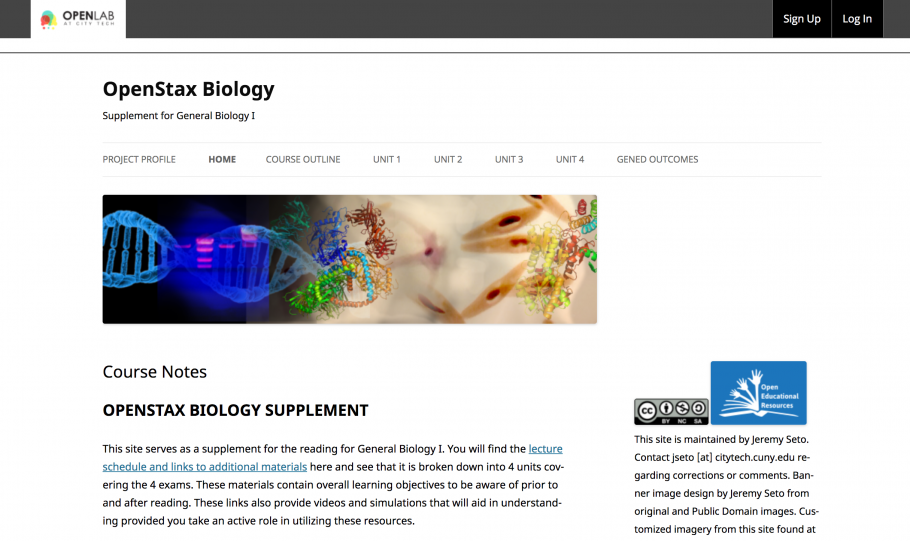The website features a predominantly black background with a white rectangle centered at the top. Zoomed in, the rectangle reveals a series of circular shapes, adorned with hair balloon icons in red, green, and yellow. Within the white rectangle, the black text reads "Open at City Tech," though the latter part becomes slightly blurry upon closer inspection. On the right-hand side of this section, white text prompts users to "Sign Up" or "Log In."

A dim, dark green line traverses the page, beneath which "OpenStax Biology" is written in black. The subtext states, "Supplement for General Biology," followed by another dim gray line. In all capital letters, the site then features a heading: "GRAZER'S PROJECT PROFILE HOME." Under this heading are units labeled Unit One, Unit Two, Unit Three, Unit Four, and Gene Outcomes.

Below this section, there is an image resembling a blue DNA molecule, with blue branches and ends in green, red, orange, and yellow highlights. Underneath the image, black text reads, "Course Notes, OpenStax Biology Supplement." A further explanation clarifies that this site serves as a supplement for reading materials in General Biology I. It includes a lecture schedule and links to additional materials, broken down into four units corresponding to the four exams.

The site emphasizes that the materials encompass all learning objectives to be familiar with before and after reading. Additionally, links to videos and simulations are provided to aid in understanding, encouraging active engagement with these resources.